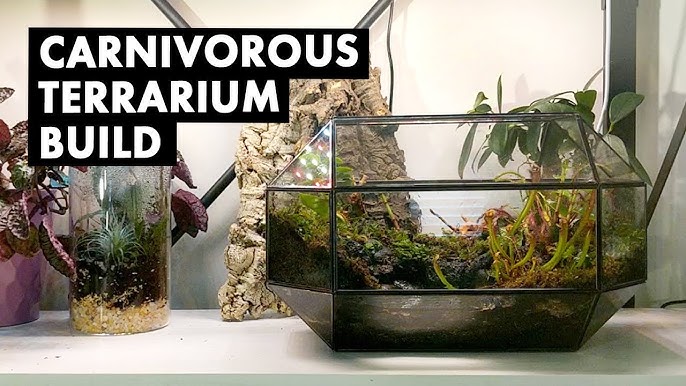The photograph captures two unique terrariums featuring an array of exotic plants. The top right side of the image displays the text "Carnivorous Terrarium Build" in white against a black background. 

On the left, there is a hexagonal (possibly octagonal) container with its base in a dark shade. The top and bottom facets are longer than the other sides, and one facet facing the camera is open, revealing an interior filled with soil, plants, and rocks. These plants appear exotic and intricate, rooted in the soil within this geometrically shaped glass vessel.

To the right, a cylindrical glass or acrylic terrarium stands tall, containing layers of substrate, with possible wooden chips or gravel at the bottom, followed by soil, and plants growing from the top. Condensation is visible on the walls of this terrarium, indicating a humid environment conducive for plant growth. Additionally, a pink vase with plants sits alongside these terrariums, and a wooden or fossilized sculpture is situated behind the cylindrical container, adding to the overall aesthetic of the scene.